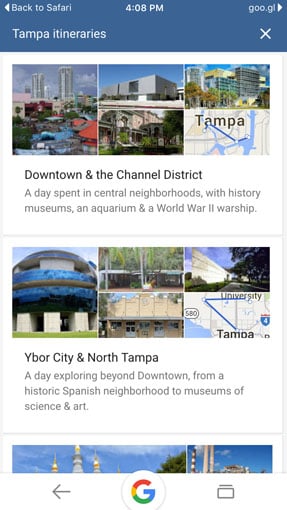The rectangular portrait image, resembling the dimensions of a cell phone screen, is more than twice as high as it is wide. It provides information about places to visit in Tampa, Florida. 

The top of the image features a slightly dark blue header with white text split into two rows. In the upper left corner, there is a filled leftward-facing arrowhead and small text that reads "Back to Safari." Centered at the top is the time, "4:08 p.m." In the upper right corner, white text displays, "GOO.GL" followed by a rightward-facing filled arrowhead. 

The second row under the header has slightly larger text. On the left, "Tampa Itineraries" is displayed, and on the right is a white "X," which appears to be a button for closing the page. 

Beneath the header, the main section of the image has a white background framed by gray borders on the sides. Near the top, there is a collage of images arranged in a 3x2 grid. The left column contains a single landscape-oriented image of Tampa’s downtown from a distance. The middle column has two stacked images: the upper one showing what appears to be a gray building, possibly an art gallery or museum, and the lower one depicting a neighborhood with brick-faced buildings and abundant greenery. The right column comprises two images as well: the lower one is a map of Tampa featuring major roads and waterways, and the upper one seems to capture a neighborhood, possibly a historic district.

Below the images, there is text with headers indicating different areas of Tampa. The first section is titled "Downtown and the Channel District" followed by descriptive text: "A day spent in central neighborhoods, with history museums, an aquarium, and on a World War II warship."

After some white space and a gray line divider, the next section is introduced with the header "Ybor City and North Tampa." The accompanying text reads: "A day exploring beyond downtown, from historic Spanish neighborhood to museums of science and art."

Another divider line appears below this, indicating the start of a third section, though it is partially cut off and mostly shows sky-filled images. The footer of the image features a white background with Google’s colorful "G" logo in the center, a leftward-facing gray arrow on the left, and a gray rectangle with a top gray line on the right.